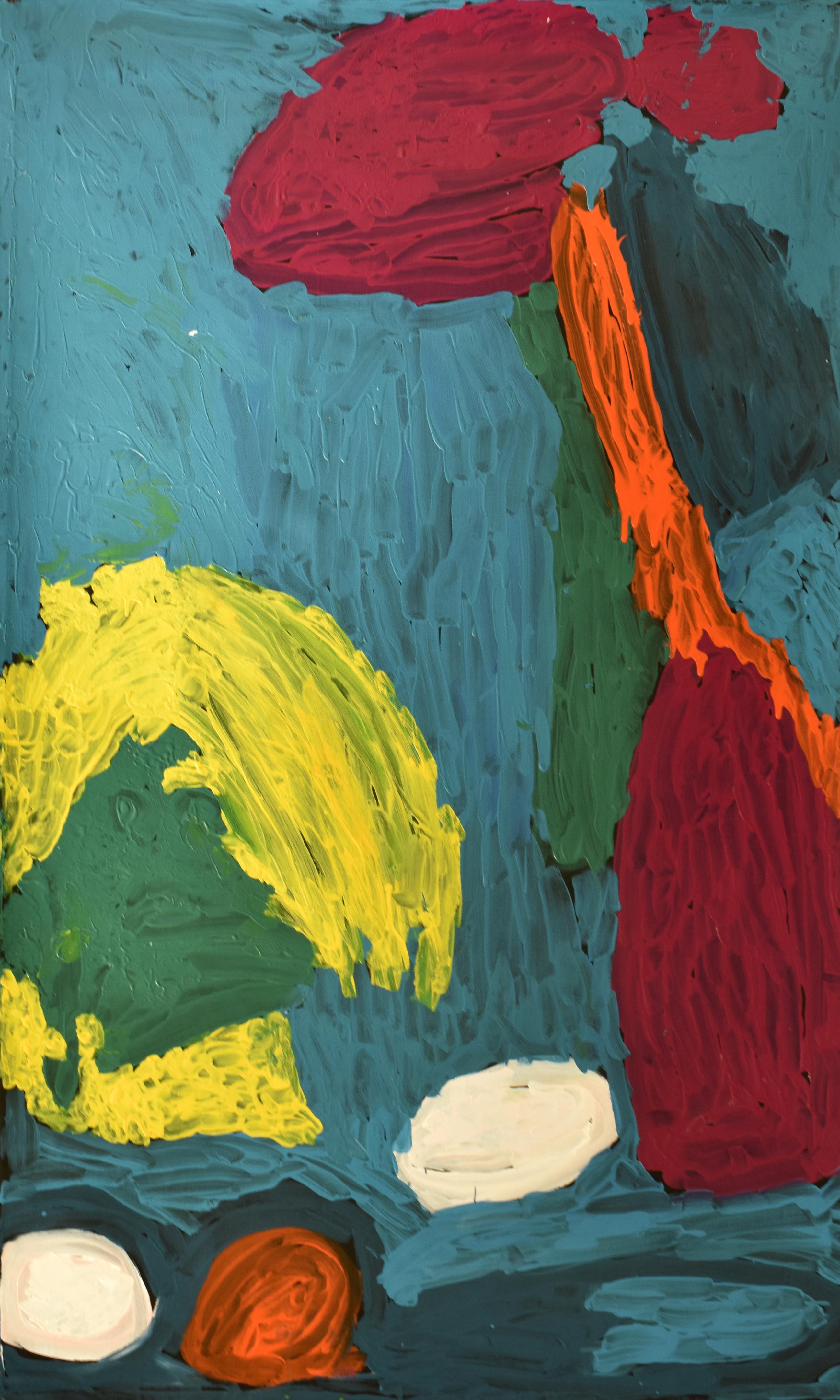The abstract painting bursts with vibrant, random shapes and dynamic brushstrokes on a light blue background. Each brushstroke is distinctly visible, underscoring the artistry involved. Dominating the right side, a red triangular shape melds with an orange pole-like form. Adjacent to these, a long, dark green sliver complements a dark blue triangular shape. A circular, heart-shaped red splotch nests above the orange sliver. In the bottom middle, a white splotch stands out, while the bottom left corner features layered oval shapes in white and orange, topped with a yellow splotch encircling a green center. Yellow paint radiates around a round green splotch on the left, adding a burst of brightness to the composition. The painting exudes a sense of chaotic harmony through its thick, tactile streaks of color and abstract forms that intriguingly suggest vague, familiar shapes without depicting anything concrete.